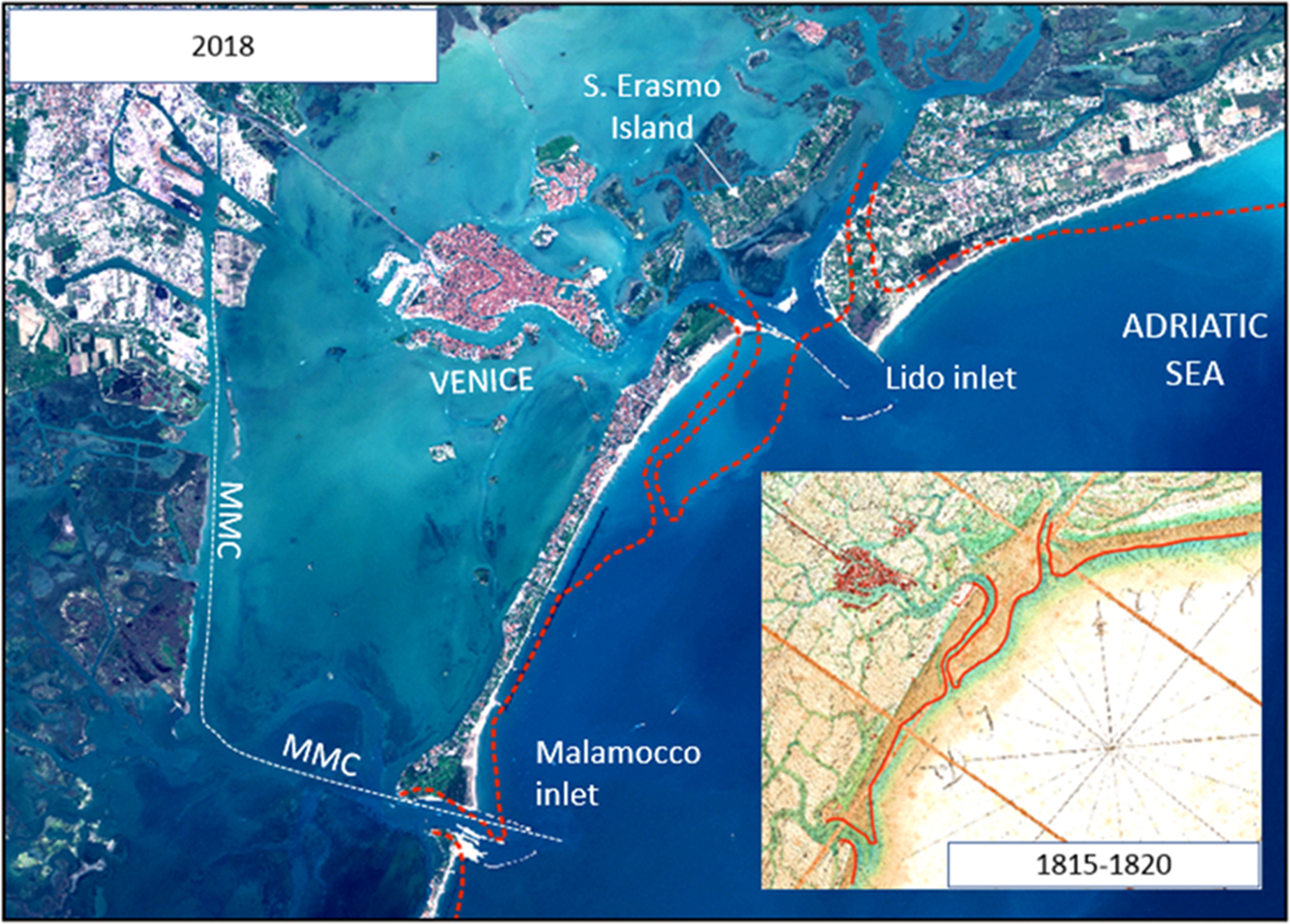The image is an aerial photograph, taken in 2018, depicting the Venetian Lagoon and its surroundings, including Venice, St. Erasmo Island, Lido Inlet, the Adriatic Sea, and Malamoco Inlet. The main photo, positioned against a white background with the year "2018" marked in black numbers in the top left corner, shows a series of red and white dotted lines indicating geographical changes over time. In the bottom right corner, there is a smaller, colorful cartographic map that dates from 1815-1820, providing a historical comparison that highlights the differences in the landscape and mapping of the region. Venice appears densely populated in the modern image, showing the shifts and modifications that have occurred over the centuries. The detailed view, possibly taken from NASA, offers a comprehensive overview of the islands and surrounding waters, illustrating the evolution of this iconic area.